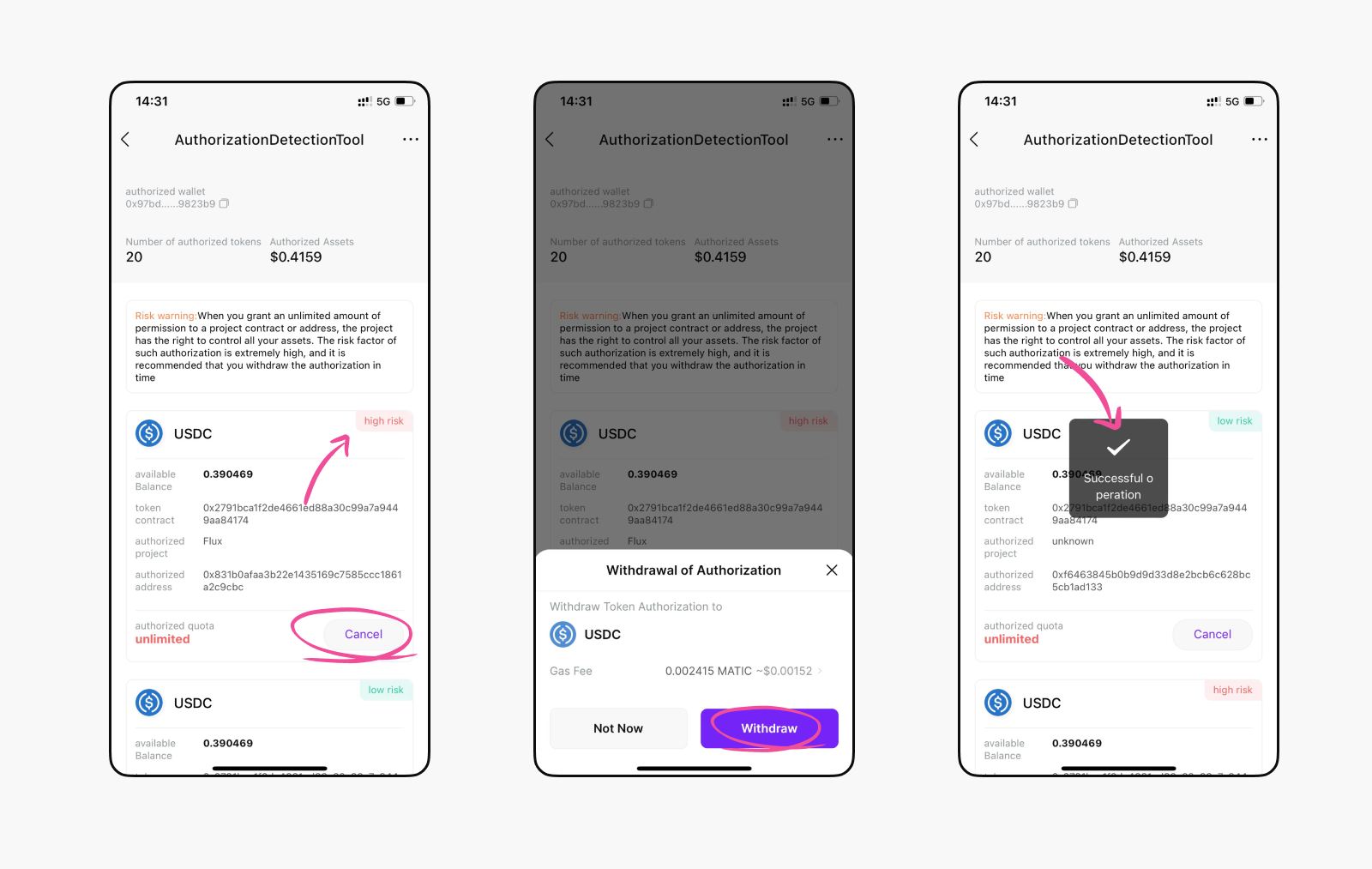The image series consists of three screenshots from a cellphone, each against a white background. The first image displays a tool titled "Authorized Detection Tool," featuring several interactive elements. It includes a round Cancel button, which appears in a blue or purple hue. There's a line extending from a long token contract number, culminating in a "High Risk" indicator on the right side, marked by a pink button with red text.

In the second image, the screen is overlaid with a gray film, bringing focus to a white, rectangular pop-up window. The pop-up is titled "Withdrawal of Authorization," accompanied by a close (X) button. It details an option to withdraw token authorization for USDC, showing gas fees of 0.0024 and 0.0015. At the bottom, there's a withdrawal button, also in a shade of blue or purple, encircled conspicuously in red.

The third image presents a risk warning message: "When you grant an unlimited amount of permission to a project contract or address, the project has the right to control all your assets. The risk factor of such authorization is extremely high, and it is recommended to withdraw the authorization in time." Below this message, a gray box pops up, displaying "Successful Operation" with a check mark. A red arrow is drawn from the warning message to the success notification, emphasizing the importance of the operation.